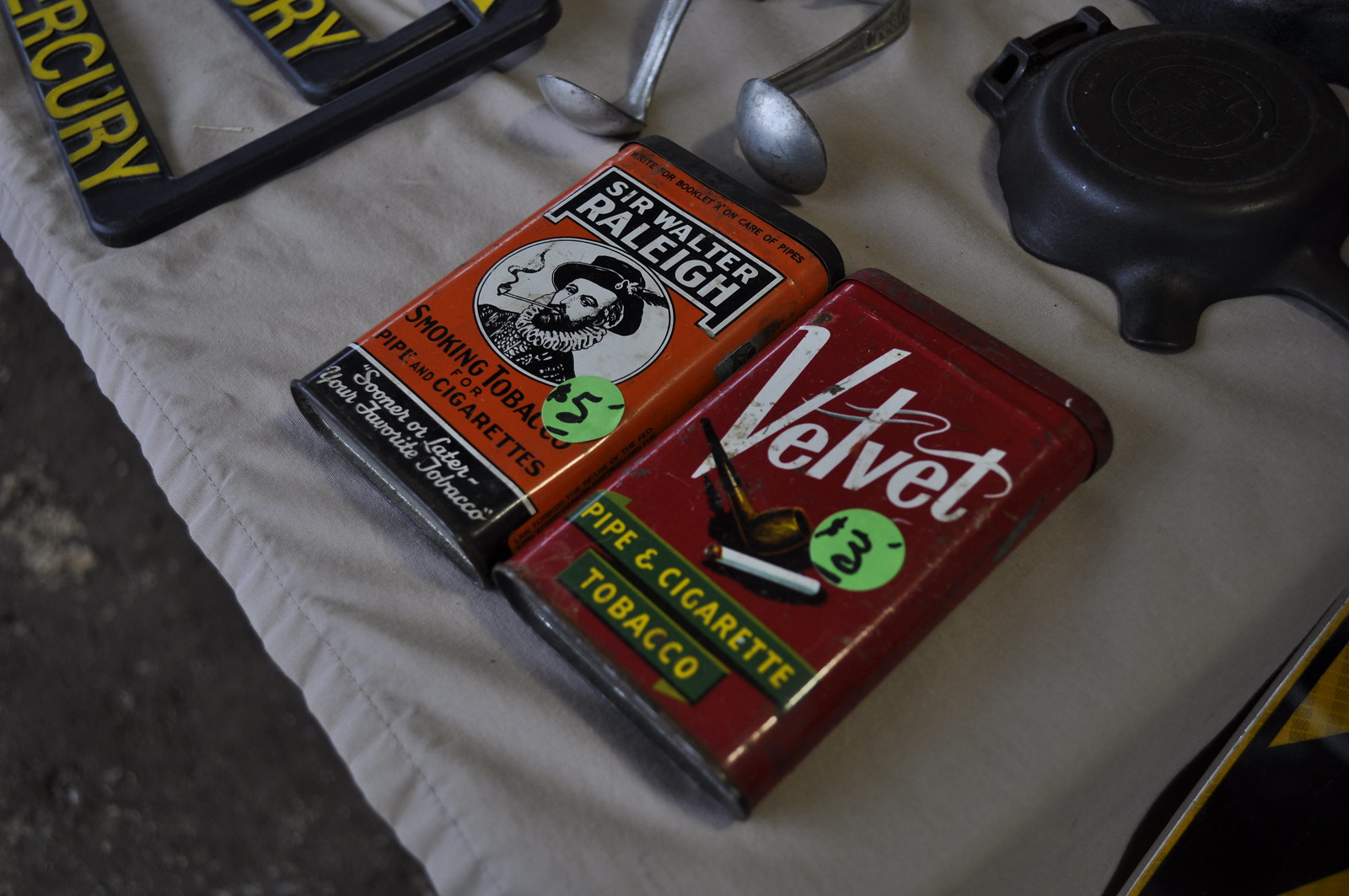The image is a color photograph, depicted in a landscape orientation, focusing on two vintage cigarette tins placed diagonally on a white tablecloth. The first tin, positioned on the upper left, is orange with bold lettering that reads "Sir Walter Raleigh" in white on a black background. Below this is a circular portrait of Sir Walter Raleigh himself, smoking a pipe, rendered in black and white line art. The tin further describes the contents as "smoking tobacco for pipe and cigarettes" and is marked with a price of $5.

To the right, the second tin is dark red, featuring the brand name "Velvet" in prominent white script across the top. Beneath, there is an illustration of a lit cigarette, and the description "pipe and cigarette tobacco" in yellow letters on a green strip. This tin is priced at $3. Both tins are surrounded by other vintage items, including two metallic spoons in the upper middle, a black gas cap in the upper right corner, and seemingly stacked license plate frames with the letters "E-R-C-U-R-Y," likely spelling "Mercury." The overall image captures these items with photographic realism, detailing their nostalgic and historical charm.